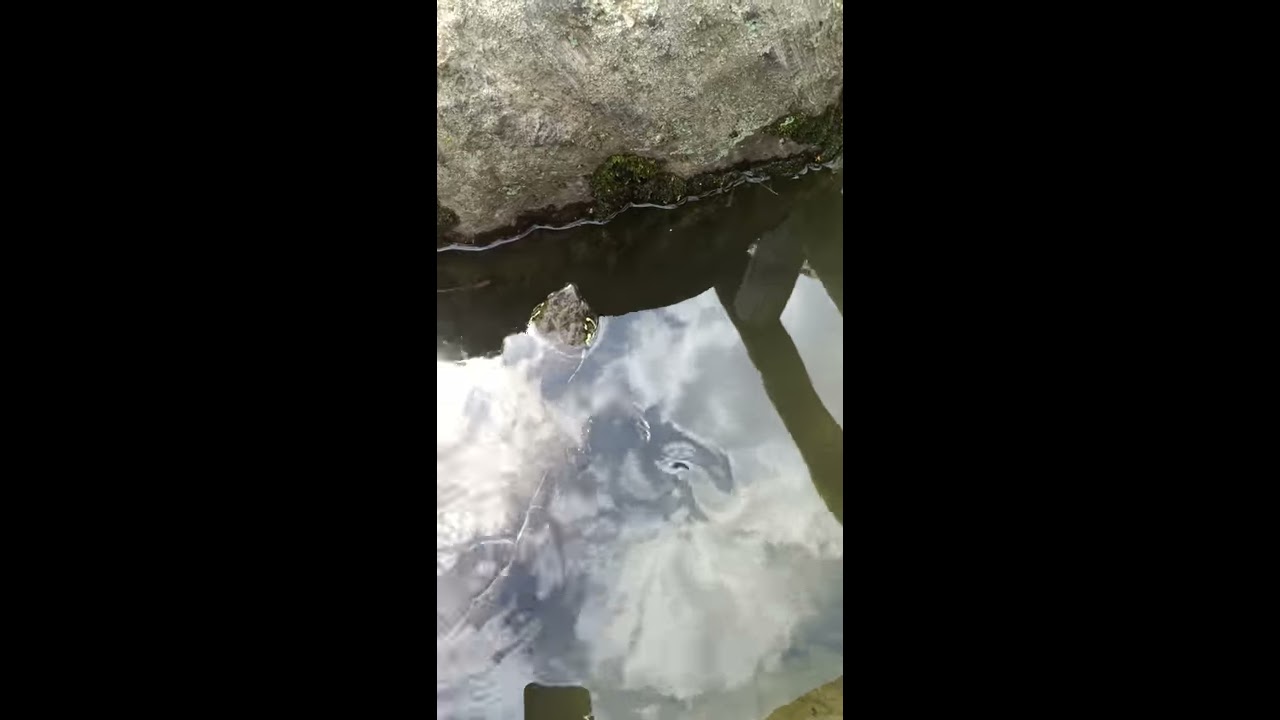This image is a horizontally aligned rectangular picture with thick, black vertical rectangles on both sides, creating wide borders. In the middle, there's a narrower vertical rectangular image that seems to depict an outdoor scene. At the top of this central image, there's a textured gray and white stone with smooth areas and a hint of green moss on its side. A thin white line demarcates the top and the side of the stone. Beneath the stone, a swirl of gray and white hues resembling clouds or possibly water creates a dynamic pattern. The scene appears to involve a pond or shallow body of murky, reflective water with shades of green. Emerging from the water on the left side is a turtle, identifiable by its dark green skin and yellow eyes, with a bit of its shell visible just below the surface. The overall setting is somewhat ambiguous, evoking elements of both the sky and water.